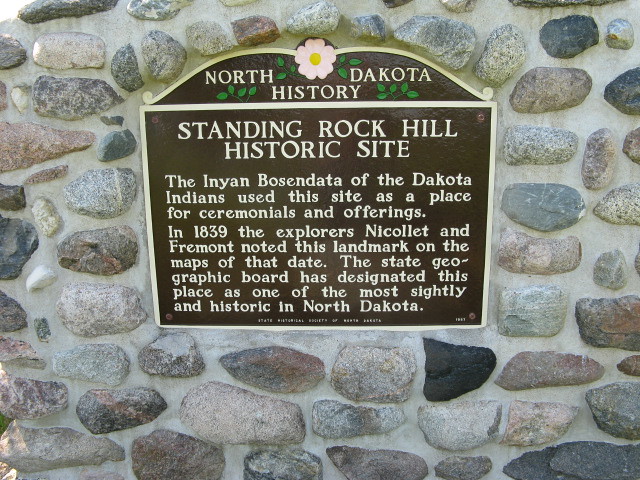In the center of the image, a detailed plaque is mounted on an intriguing cemented wall adorned with various small, round rocks reminiscent of a cleaned brook bed. The wall, evoking an aged Victorian or English style, enhances the historic ambiance of the scene. Positioned on this unique wall, the plaque features a dark brown background with gold lettering and a curvaceous top framing a pink flower with green leaves.

The top of the plaque reads "North Dakota History," followed by "Standing Rock Hill Historic Site" in a rectangle below. The plaque details that the Dakota Indians used this site for ceremonies and offerings, and highlights that in 1839, explorers Nicollet and Fremont recorded this landmark on their map. The State Geographic Board has since recognized it as one of the most scenic and historic locations in North Dakota. The colors in the scene include white, gray, tan, brown, black, green, and yellow, all indicating an outdoor setting during daylight in a historic area.